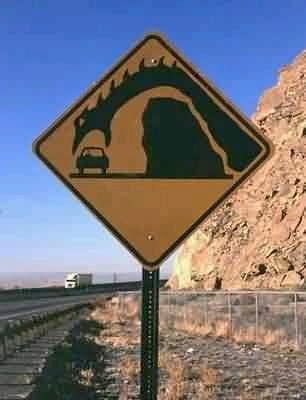The image showcases a diamond-shaped street sign with a vivid yellow background and a black border. The sign depicts a fantastical scene where a dragon is stretching its neck over a mountain to capture a car, suggesting that it may be a fictional or digitally created sign. In the background, a roadway is visible, which initially resembles railroad tracks but is confirmed as a road due to the presence of a large white 18-wheeler truck approaching from the distance. To the right of the roadway, the landscape transitions into a desert-like terrain featuring rocks, sand, and sparse dead vegetation. The scene is framed by a prominent rocky mountain on the right side of the image and a clear blue sky overhead.